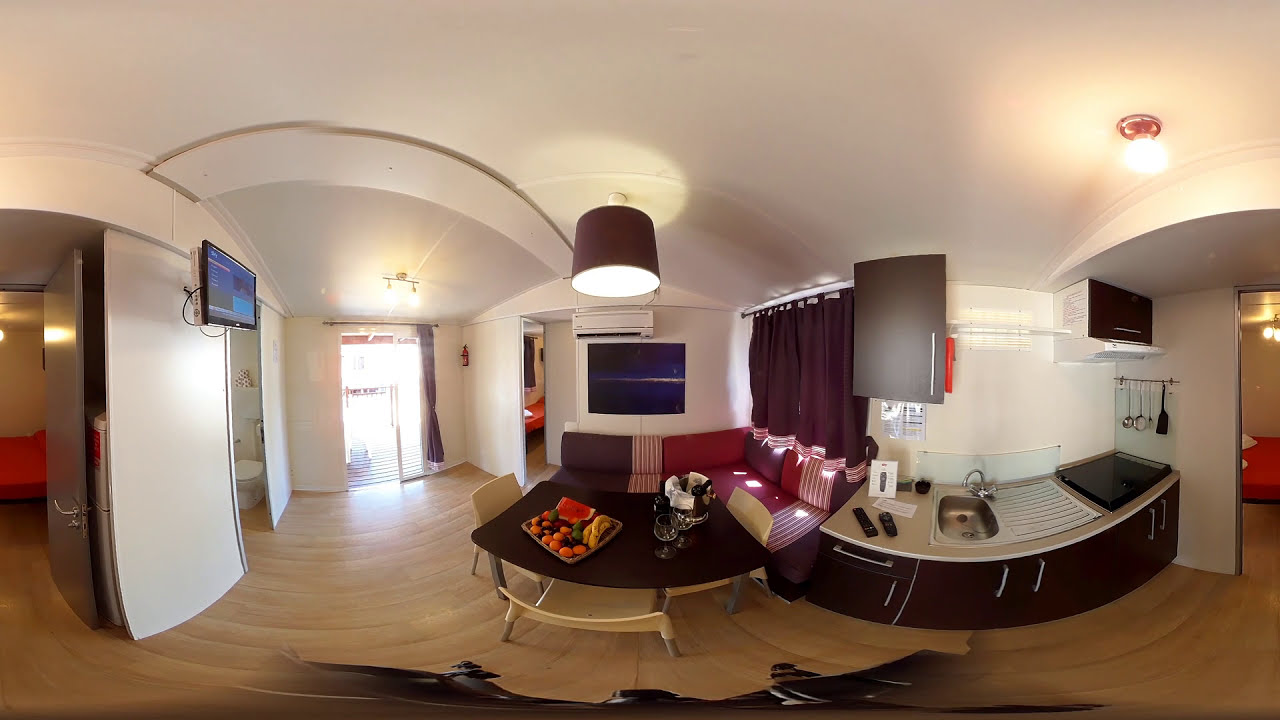The image depicts the interior of what appears to be a living room in an apartment or an Airbnb-style rental, captured in a daylight photograph with a slightly panoramic view. The room features polished light wood flooring and white walls and ceiling. At the center left, there is an arched glass doorway that allows sunlight to stream into the space. Overhead, a central light with a dark brown lampshade is suspended above a seating area consisting of an L-shaped couch adorned with red and striped vertical brown and tan cushions. A curved coffee table is positioned in front of the sofa. 

To the right, there is a curved countertop leading into what seems to be a kitchen area equipped with a microwave, stovetop, sink, and dark-colored cabinets. Above this counter, a gray metal cabinet is mounted on the wall, under which various devices, possibly a charging station, are situated. Adjacent to this area is a dining table with a tray of fruit, including tangerines, watermelon, and bananas.

A flat-panel TV is mounted on the wall behind the sofa. On the far left of the image, there is a partially visible partition with a red chair, hinting at another room. An entry to a bathroom is located on the left side, with a high-mounted TV just before it. Sliding doors near the center likely lead to a patio, and thick curved molding elegantly frames various transitions between spaces, adding architectural interest. The photograph captures a cozy yet meticulously arranged living environment, possibly intended for rental purposes.